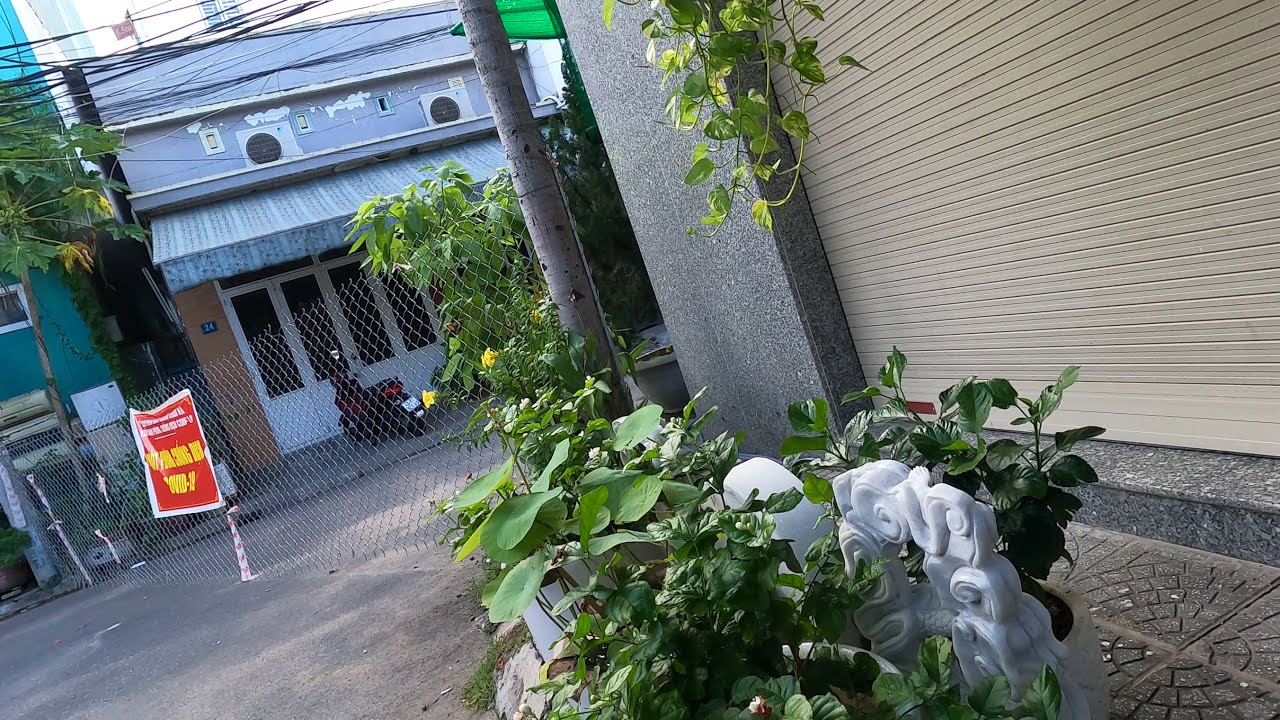This image is a detailed color photograph of an outdoor city scene, seemingly in Japan. It captures the exterior corner of a building with a closed, tan-colored garage-style door against a backdrop of gray slate siding. In the foreground, there are numerous potted green plants with intricate, ornate carved stone backgrounds and some flower beds. Among these, a couple of yellow flowers can be seen mingling with the green leaves. Additionally, a tree stands beside the building, its gray trunk prominent amidst the greenery, and a hanging plant with long stems adorns the wall. To the left, the scene extends into a street flanked by buildings, the road partially obstructed by a chain-link fence. Suspended on this fence is a red sign with white and yellow text, likely in an Asian script. Power lines stretched across the top left corner of the image add a subtle urban touch to the tableau.